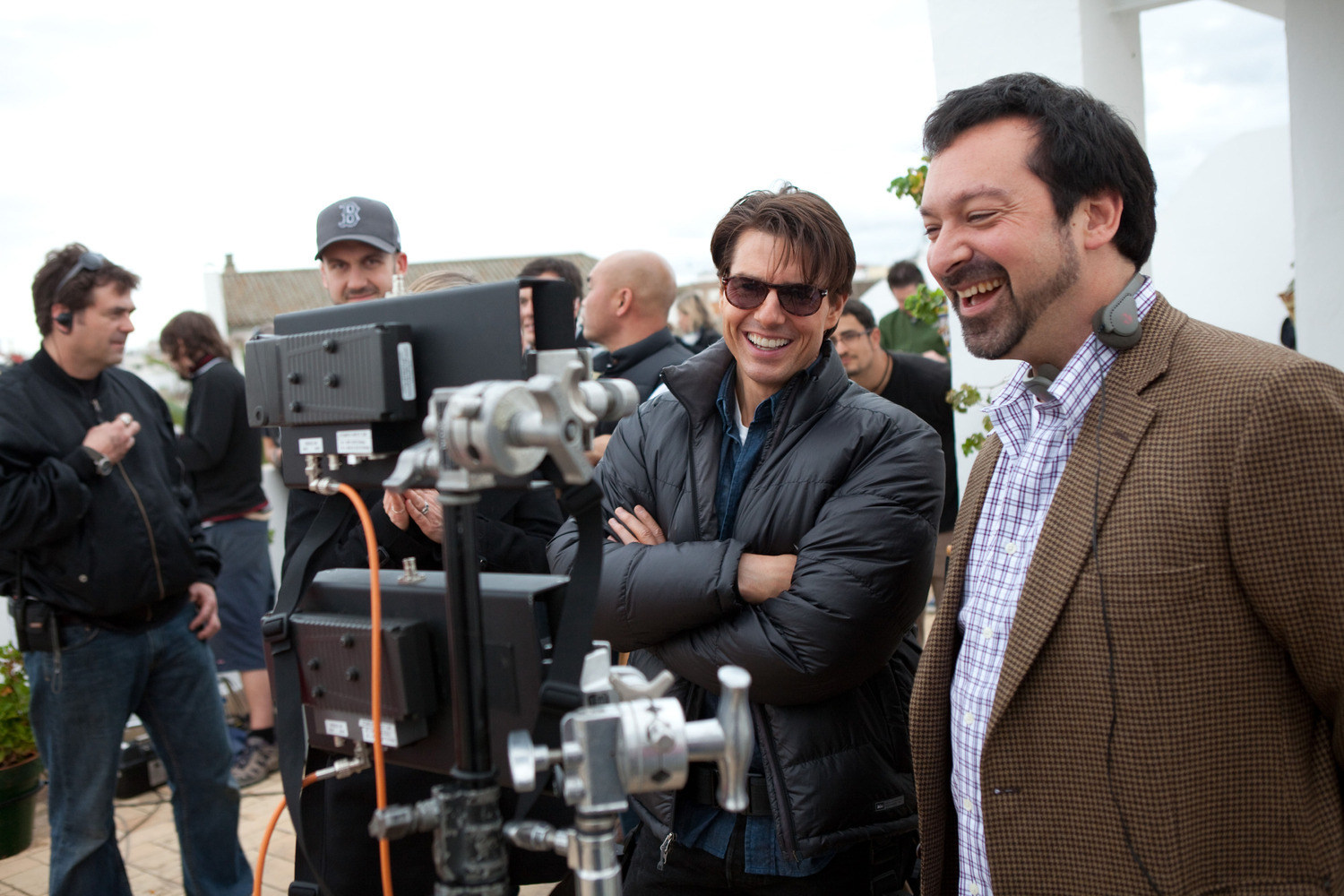The image captures a bustling film set, likely during a daytime shoot, featuring a mix of earthy and neutral colors including beige, tan, black, brown, blue, and white. At the center of the image is Tom Cruise, recognizable by his black puffy jacket and dark sunglasses, engaged in a light-hearted moment alongside a man to his right. This man is wearing a checkered shirt and brown checkered jacket, with headphones around his neck, and is laughing while both actors focus on a set of monitors in front of them, likely reviewing recent takes. Behind them, numerous crew members mill around, engaged in various activities, with the setting resembling an exterior location possibly near a terrace or building visible in the distant background. The overall scene conveys a lively yet professional atmosphere typical of a movie set between takes.